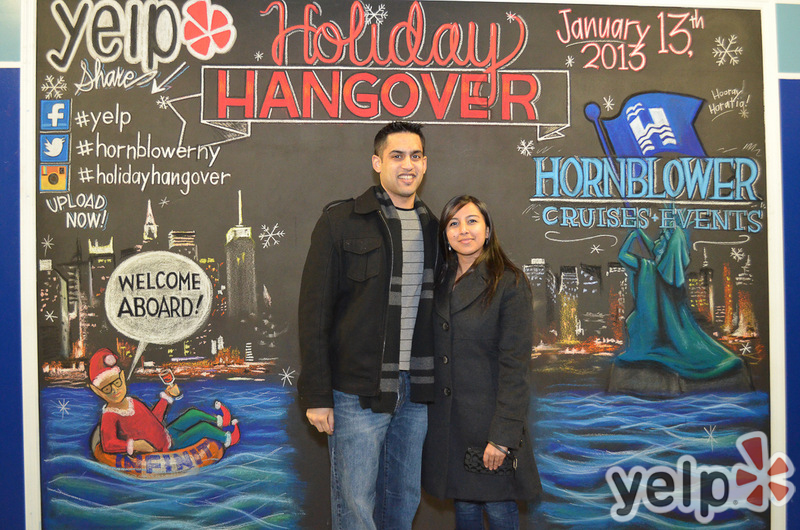In this image, a young Hispanic couple dressed casually in coats stands in front of a vibrant promotional billboard for Yelp. The billboard announces the "Holiday Hangover" event in striking red text, with a clever snowflake dotting the "I," set against a nighttime city skyline. The event date, January 13, 2013, is displayed prominently in white text on a red background. Below the event information is blue text saying "Hornblower Cruises and Events," accompanied by a logo featuring the Statue of Liberty blowing a horn with a blue flag. 

To the left, social media icons for Yelp, Facebook, Twitter (@HornblowerNY), and Instagram are displayed alongside hashtags #HolidayHangover and #HornblowerNewYork. Adding a whimsical touch to the scene, an elf in costume sits on a life raft to the left of the couple, holding a drink with a playful "Welcome Aboard" caption nearby. The background is adorned with snowflakes, enhancing the festive atmosphere. The man, with a big smile on his face, wears a black jacket, blue jeans, and a gray and white shirt, while the woman beside him sports a long gray coat and blue jeans, her long brown hair framing her cheerful expression.